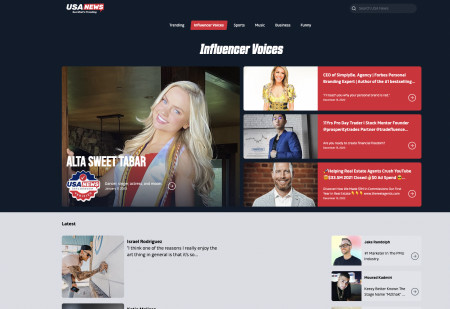The image depicts a segment from a U.S. news website with a notably low resolution. The background is a dark blue, almost black, color. In the upper left corner, the text "USA News" is prominently displayed, although the text below it is illegible. To the right of this header, there is a search bar.

Beneath the search bar is a white navigation menu containing five links, with one of the links enclosed in a red rectangle with horizontal orientation, featuring white text that is difficult to discern. Directly below this navigation menu, the section titled "Influencer Voices" showcases a photograph of a fair-skinned, blonde woman with blue eyes, identified as "Alta Sweet Tabar, U.S. News."

Adjacent to her photo, there are three additional individual photographs, each accompanied by a red bar with white text, which is unreadable. The background remains consistently dark blue/black throughout this segment.

At the bottom of the image, there is a grey strip featuring three photographs: a large one on the left and two smaller ones on the right.